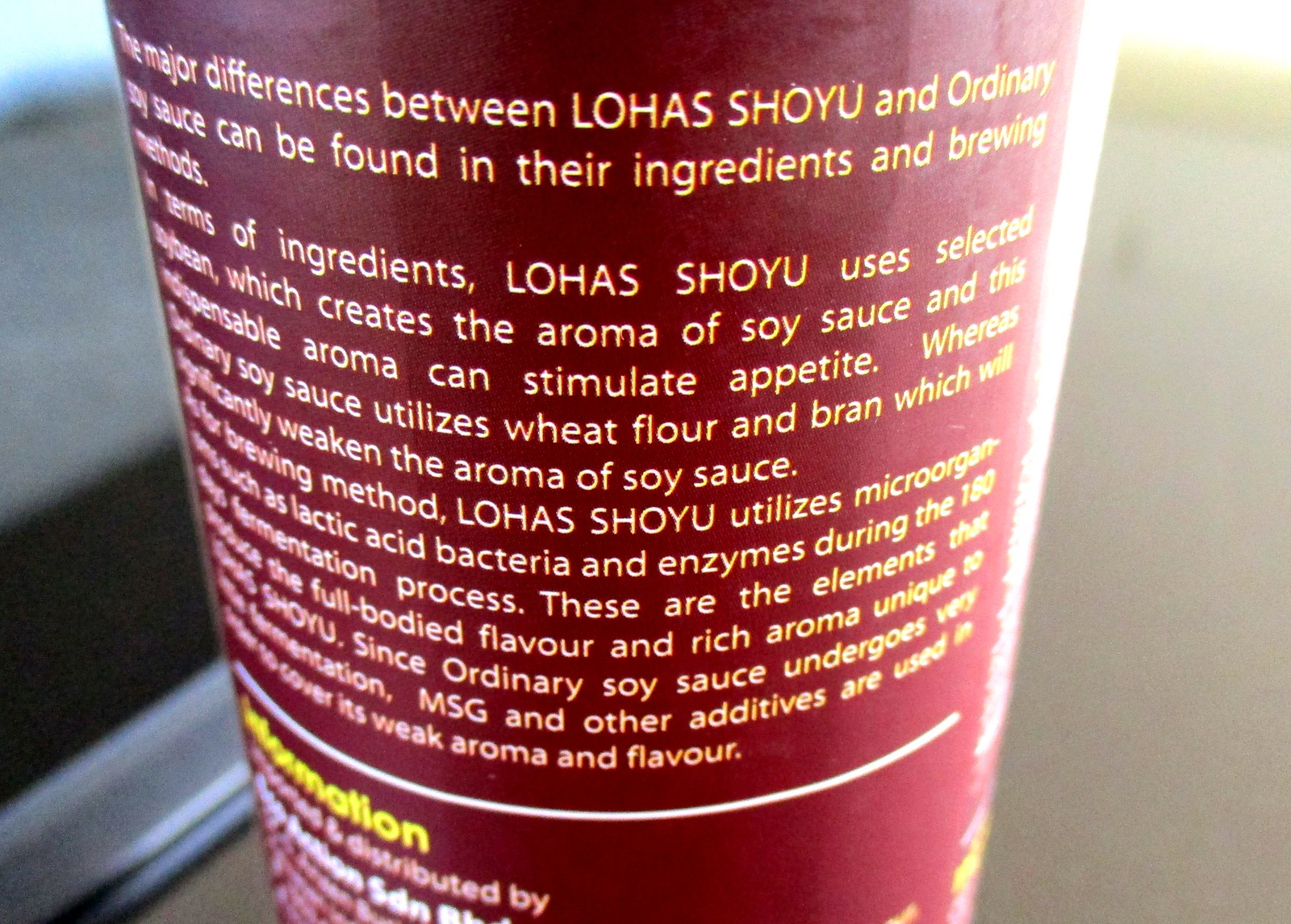This image is a close-up of the back of a soy sauce bottle with a maroon label adorned with yellow and white text. The label details the major differences between Lojas Shoyu and ordinary soy sauce, focusing on their ingredients and brewing methods. Lojas Shoyu uses selected soybeans, which create an aroma that is described as indispensable for stimulating appetite. In contrast, ordinary soy sauce utilizes wheat flour and bran, significantly weakening its aroma. The brewing method for Lojas Shoyu involves a meticulous 180-day fermentation process with microorganisms such as lactic acid bacteria and enzymes, contributing to its full-bodied flavor and rich aroma. Ordinary soy sauce, with its minimal fermentation, relies on MSG and other additives to mask its weak aroma and flavor. The bottle is positioned on what appears to be a white kitchen counter.